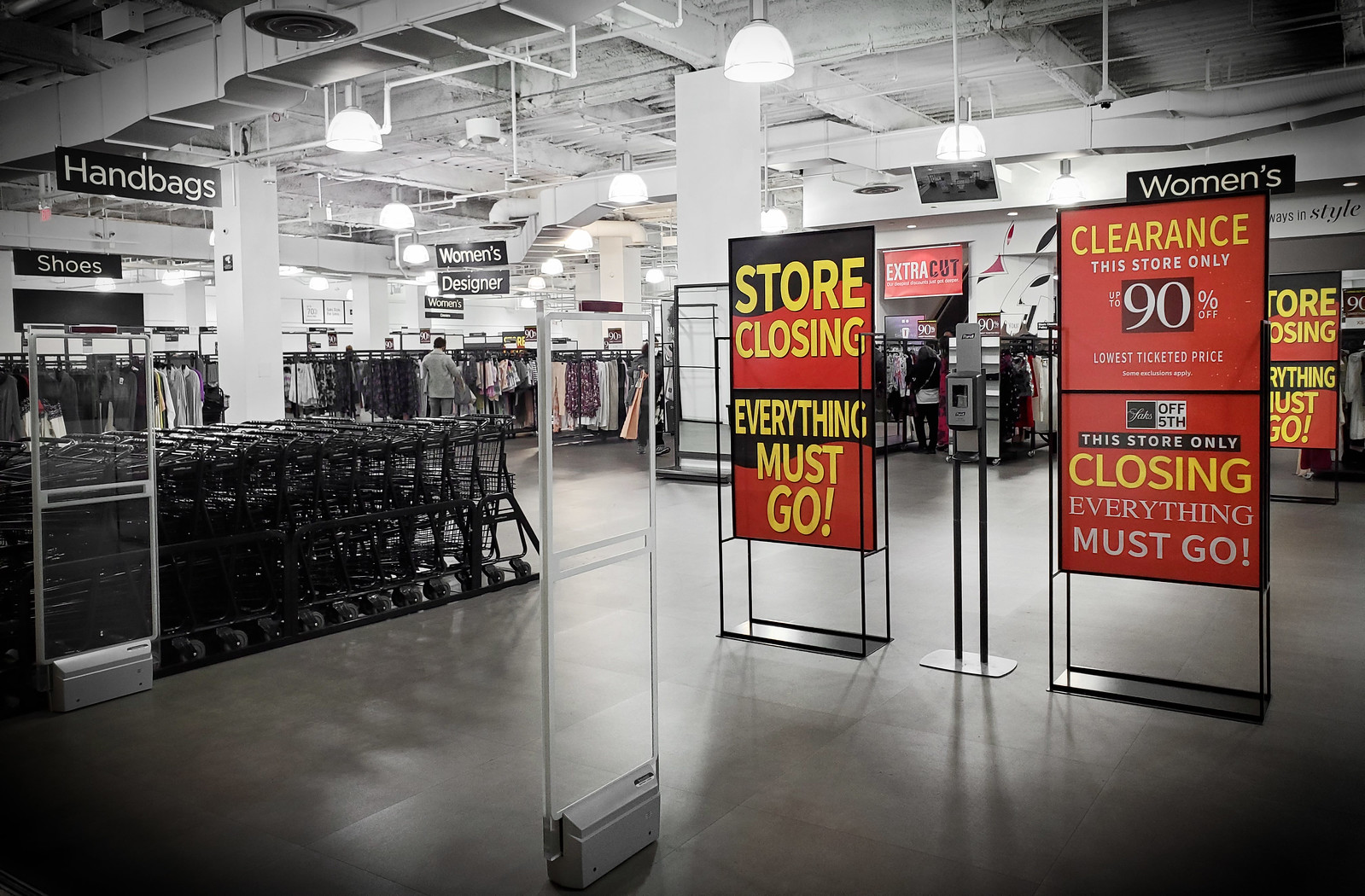The image depicts the interior of a large department store, characterized by a warehouse-like design with huge vaulted ceilings, visible piping, and metal rafters. The store is primarily shown in black and white, with the exception of several prominent signs in red, black, and yellow. These signs, two or three in total, announce an imminent store closing, with messages such as "Store Closing," "Everything Must Go," "Clearance," and "90% Off." These signs emphasize the urgency and scale of the clearance sale. On the left-hand side of the image, overhead signs indicate sections dedicated to "Handbags," "Shoes," and "Women's Designer" items. Additionally, you can see some trolley carts and scan detectors near the middle, further suggesting a retail environment. On the right-hand side, there's another sign simply labeled "Women's," adding to the focus on women's apparel and accessories. The overall atmosphere captured is one of significant markdowns and final sales in a spacious, industrial-style department store.